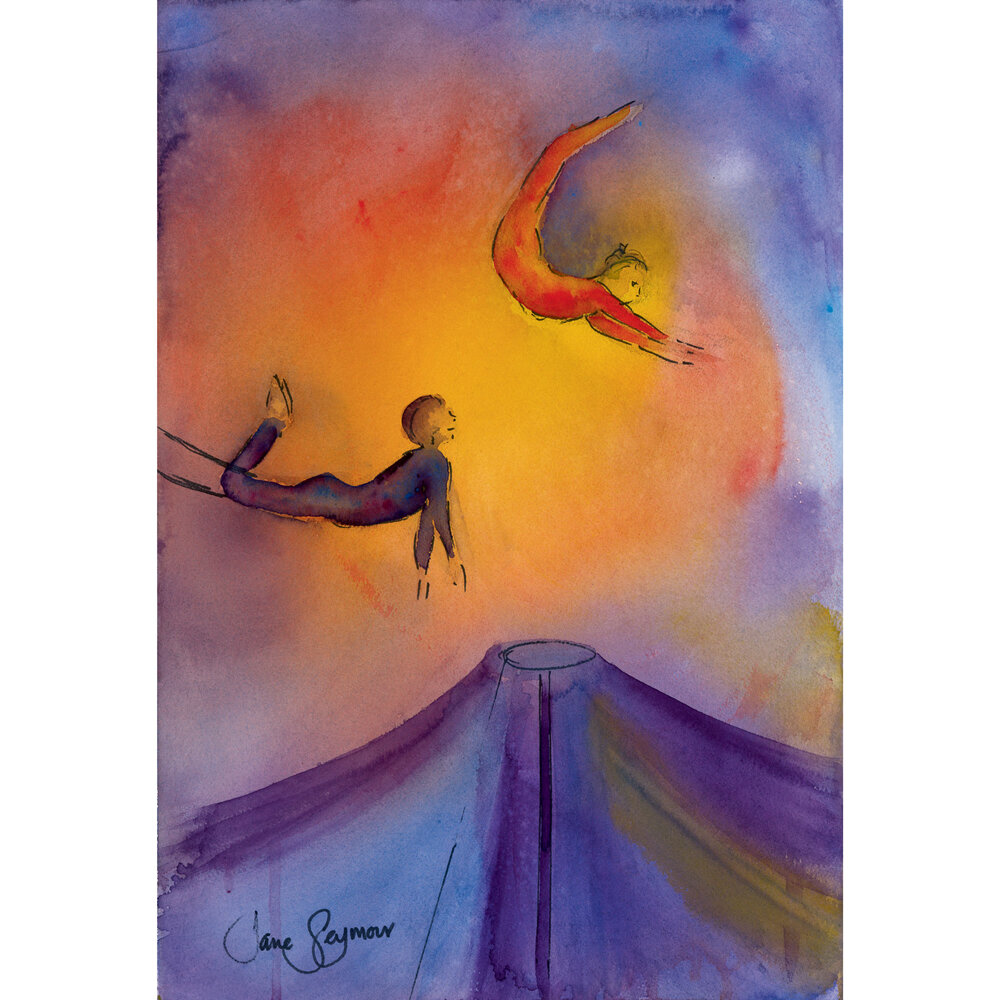This vivid painting, likely a watercolor or oil piece by artist Jane Seymour, captures a dynamic circus scene. Central to the composition are two acrobats performing mid-air maneuvers against a vibrant background of yellow, red, and blue hues. On the left, one performer, clad in blue, swings effortlessly from a rope, while on the right, another acrobat, dressed in red, contorts their body, with arms outstretched and spine arched backward. Their figures are defined by yellow tones and bold black outlines, enhancing their dramatic poses. Below them stands a large, conical circus tent shaded predominantly in purple with accents of blue and yellow. The artist's signature, "Jane Seymour," is discreetly placed in the bottom left corner, lending authenticity to this lively depiction of a carnival spectacle.